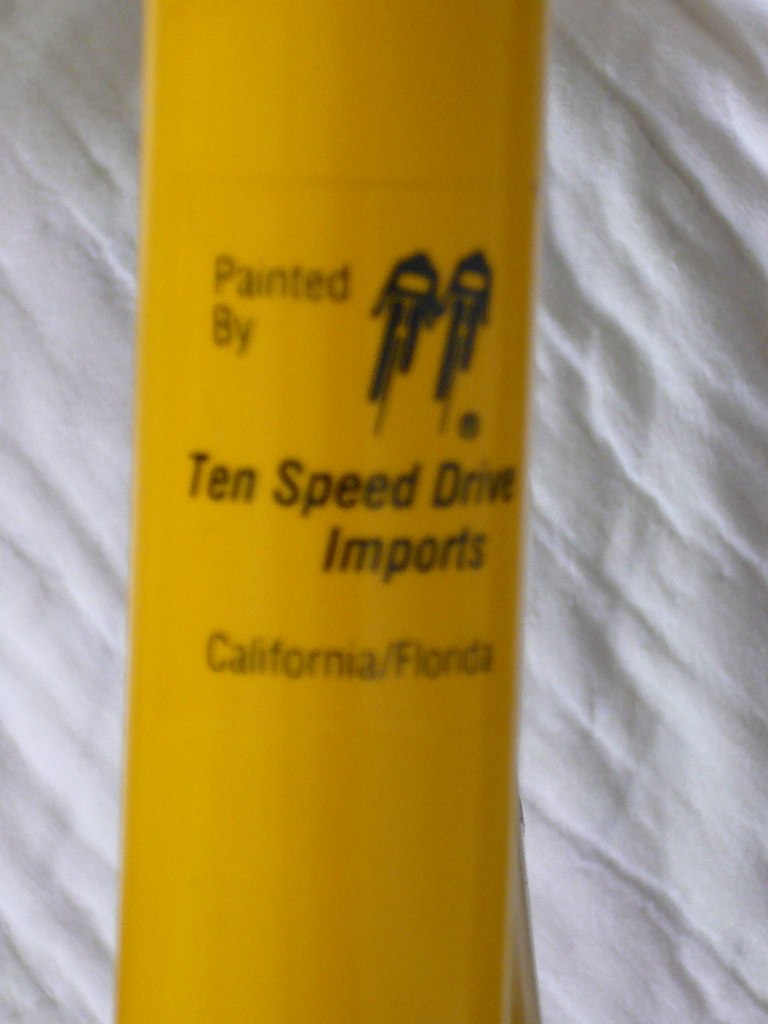In this rectangular image, a yellow cylindrical object is prominently displayed against a white cloth backdrop with diagonal creases. The object is painted in a shiny, ceramic-looking yellow with detailed black text and images. The text on the cylinder reads "painted by 10 Speed Drive Imports, California / Florida." To the right of this text are black outlines of two bicyclists in tandem, both appearing to be hunched over and possibly wearing helmets. The cylinder's purpose is unclear, but the overall scene emphasizes the contrast between the bright yellow object and the subdued white background.